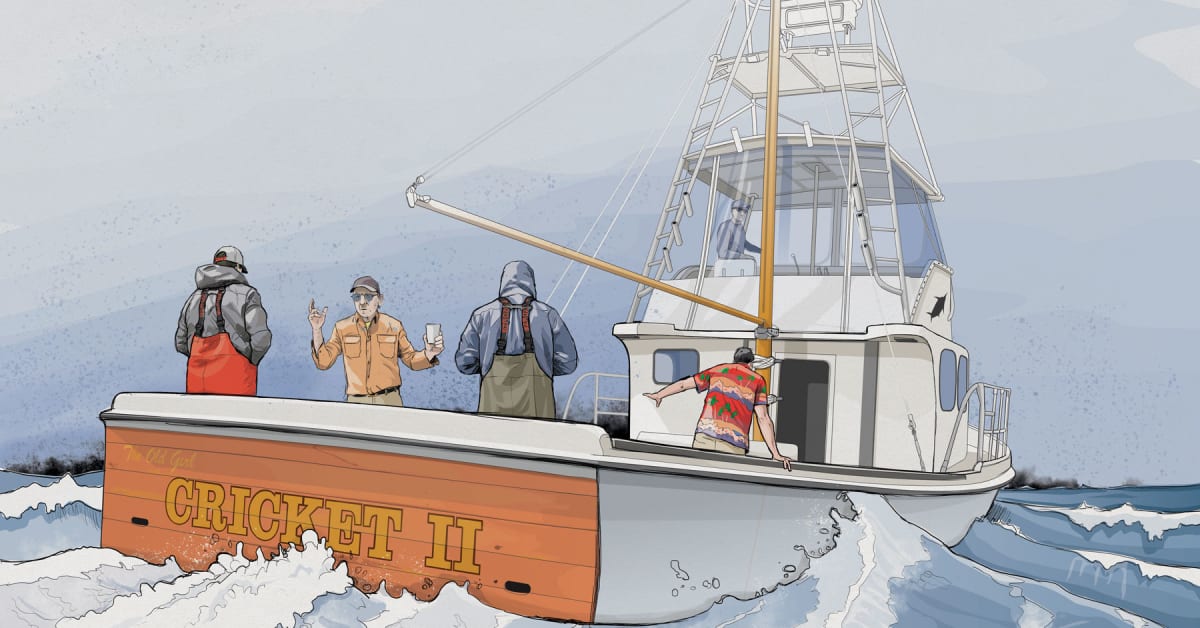In this detailed comic-style drawing, a fishing boat named "Cricket II" navigates choppy waters, conveying a sense of rough sailing. The boat, with its white body and wooden paneling featuring the name written in gold or yellow, carries five individuals. Three of these men, identifiable as seasoned fishermen by their wader-style overalls and hooded sweatshirts, seem to grapple with the adverse weather conditions. One man is clutching the rail tightly, while another appears to be attempting to enjoy a drink in the midst of the tumult. The man with the drink wears a button-down shirt, glasses, and a baseball cap, and is engaged in conversation with the fishermen. A fourth man, dressed in a Hawaiian shirt, is turned away from the viewer, seemingly off-balance. Above, in the cabin of the two to three-level boat, the captain is concentrated on steering through the rough waves. In the background, a dark, blurry presence hints at a distant fire, with ash hovering above the water, adding a layer of intensity to the scene.